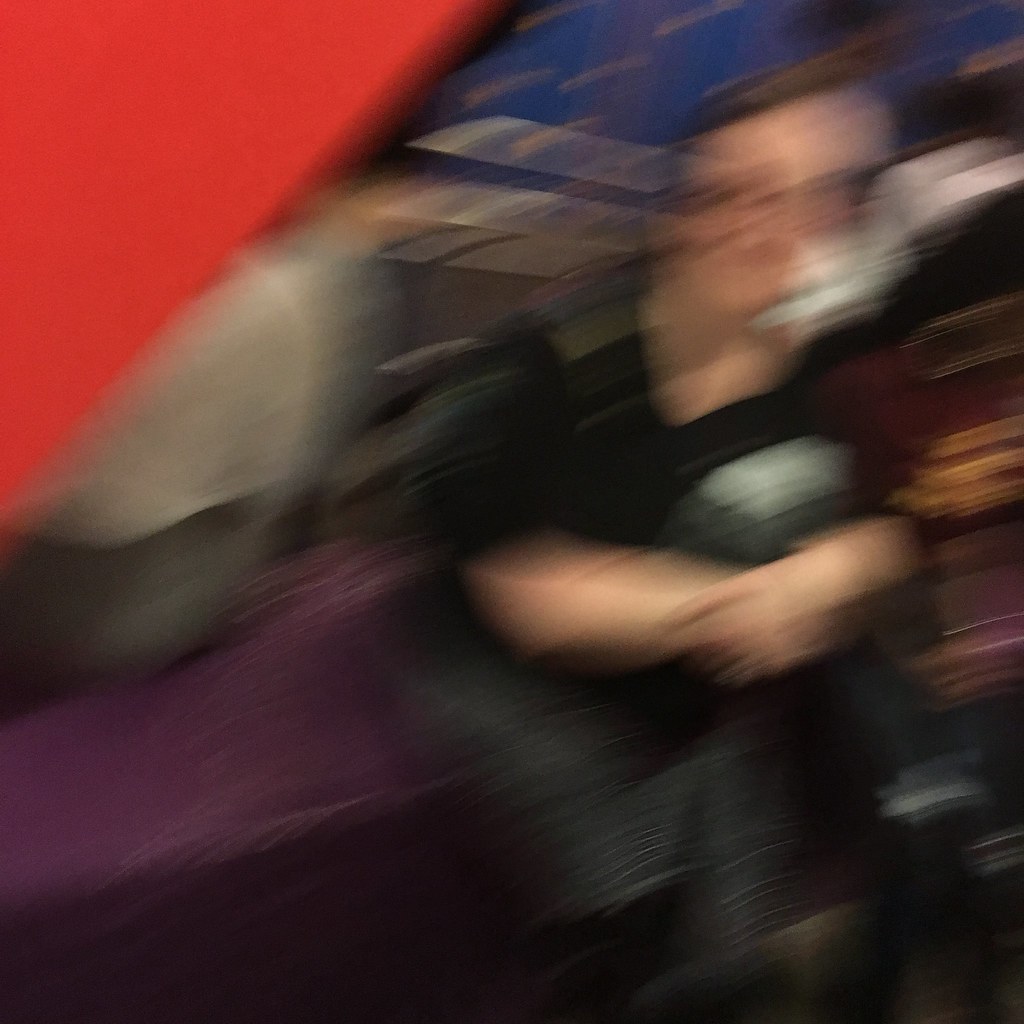The blurred image depicts a man sitting down, identifiable by his short medium to dark brown hair. He appears to be smiling and has his arms and legs crossed. He is wearing a black T-shirt and dark pants, although one description mentions blue jeans. The man's T-shirt seems to have a white graphic or writing on the upper left chest area. To his left, there is a cooler with a white lid and gray bottom, and nearby is a large red piece of cardboard or paper, partially cut off in the image. The man sits on a purple bench with a backdrop featuring blue, white, red, gray, and purple streaks, possibly due to a color filter or camera flare that intensifies these colors around him. His exact environment is indistinct, further obscured by additional brown and white blurred objects surrounding him.